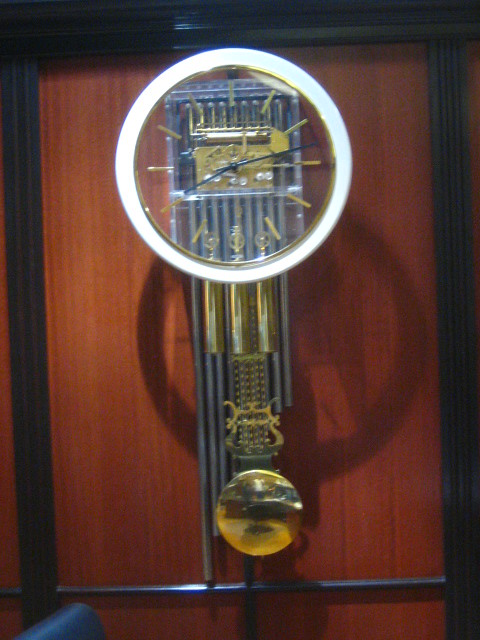This photograph captures an intricate vintage clock mounted against a wooden wall. The clock is portrayed in a vertical rectangular orientation, featuring a distinctive design. At the upper center, a prominent white circle forms the outer rim, distinguishing the clock's edge. This timepiece lacks traditional numerals; instead, it has thick, copper-colored lines that denote the hours, adding a touch of elegance to its appearance. The inner face of the clock is a clear glass, providing a glimpse of its complex inner mechanisms.

The hands of the clock are delicately thin, with the hour hand pointing towards the position where the number eight would be, and the minute hand slightly past the ten, indicating a time of approximately 8:12. Behind the clock's transparent face, one can observe an intricate silvery metal grid interspersed with coppery elements, adding depth and texture to the piece.

The background wall, composed of brown wood with vertically arranged thin grains, accentuates the clock's vintage aesthetic. The clock casts an extensive shadow towards the bottom right, enhancing the three-dimensional aspect of the image.

Emanating from the lower portion of the clock are dark gray metallic tubes that extend downwards, contributing to its antique charm. Several inches below the main body of the clock, a circular copper-colored metal disc is visible, though its purpose remains unclear. The entire ensemble is framed by a dark black border, which could be either wood or metal, creating a stark contrast against the wooden backdrop.